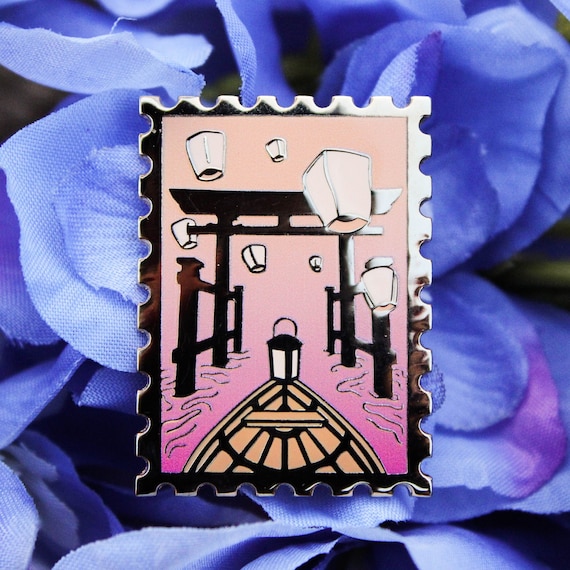The image showcases a rectangular brooch, designed to resemble a metallic postage stamp with silver perforated edges. At its center, the brooch depicts an enchanting scene where a small boat, possibly a canoe or kayak, navigates through serene pink waters, creating gentle ripples. The boat passes beneath a traditional Japanese gate or shrine structure, flanked by fences on either side. Suspended above the water are several floating, silver lanterns or containers, adding a whimsical touch to the scene. The background features an artificial flower made of synthetic material, resembling blue or purplish silk lilacs with dark gaps between the petals, lending a contrasting yet harmonious canvas to the intricate brooch.